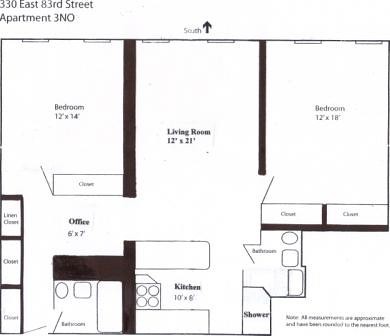Detailed overhead diagram of an apartment layout rendered on a white sheet of paper. The floor plan provides a bird's-eye view of the apartment located at 330 East 83rd Street, Unit 3NO. This is a single residential unit featuring two bedrooms, situated on the top left and top right corners of the diagram. Nestled between the two bedrooms is an expansive living room area, designed to serve as the central communal space. 

The unit boasts ample storage with two closets in the top-left bedroom and one closet in the top-right bedroom. Adjacent to the living room is a cozy office nook, providing a perfect spot for remote work or study. A spacious kitchen is situated towards the bottom of the layout, equipped to handle all culinary needs. The apartment includes two bathrooms—one large bathroom located centrally for convenient access, and another, smaller bathroom with a shower, situated near the office space. 

Each detail of the apartment—including all doors, hallways, and architectural features—is meticulously illustrated in this top-down view, making it an ideal reference for potential tenants seeking a clear understanding of the unit’s layout and room dimensions. It also serves as a valuable resource for architects and designers aiming to replicate or reconfigure the apartment’s efficient design in future projects.